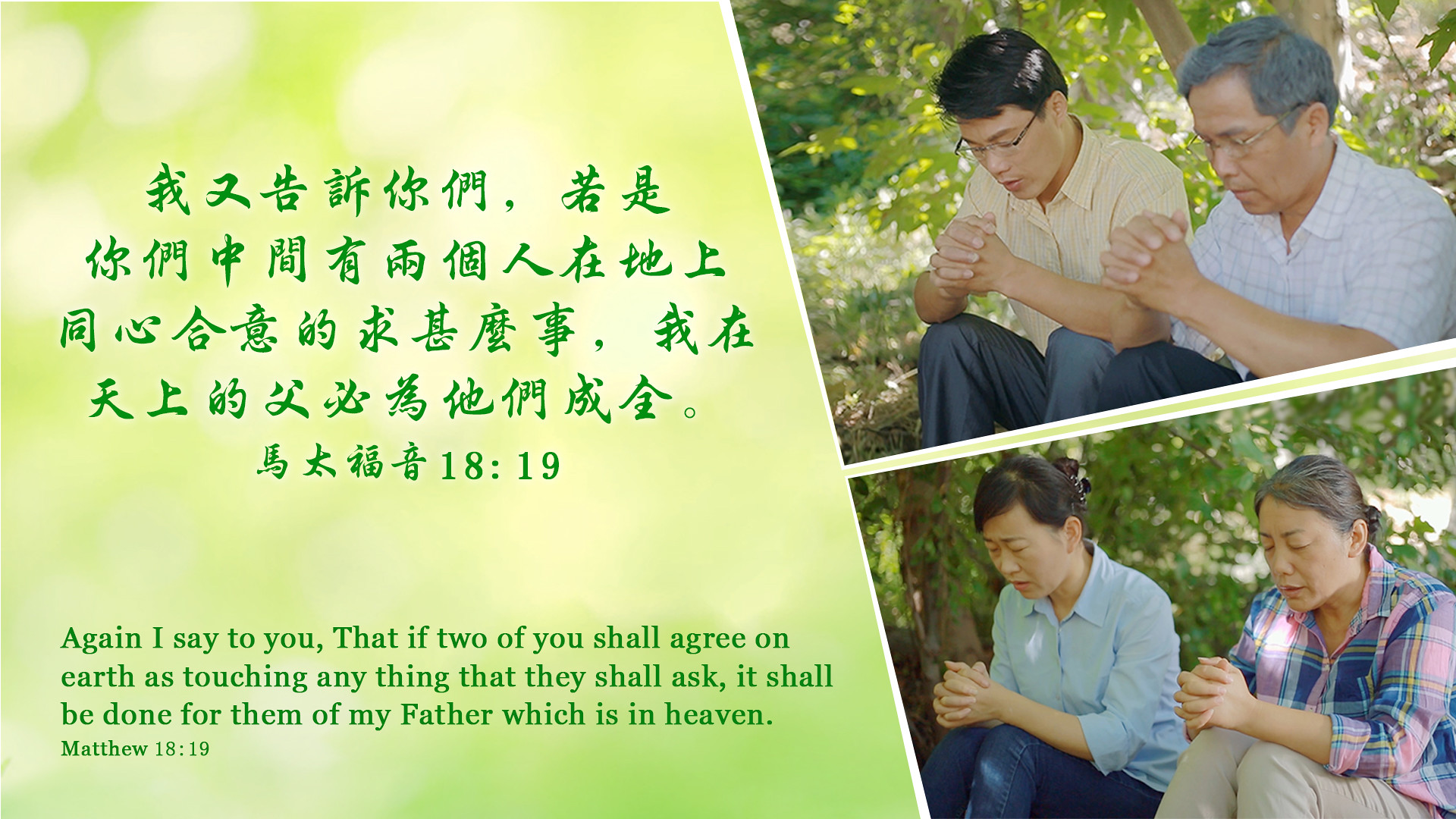The image is a horizontally aligned rectangular poster with a green-dominant background that has accents of white and yellow, evoking an outdoor setting with trees. The left side of the poster features text, while the right side showcases two diagonal images, one above the other.

On the left, there is a split effect with five centered lines of text in an Asian language, likely either Japanese or Chinese, featuring symbols with the reference "18:19" at the end. Below this, in green English text, it reads: "Again I say to you, that if two of you shall agree on earth as touching anything that they shall ask, it shall be done for them of my Father which is in heaven." A smaller print underneath attributes this quote to "Matthew 18:19."

The right side has two images. The top image depicts two Asian men, probably a 20-year-old son and his father, both dressed casually; the son in a yellow top and black slacks, and the father in a white patterned top. They are praying, with heads bowed and hands clasped. The background here includes green and yellow foliage, hinting at an outdoor setting. The bottom image shows two women, also engaged in prayer with their heads bowed and hands clasped. The woman on the left wears a light blue collared shirt and blue jeans, with dark hair pulled back in a clip, while the woman on the right sports a pink and blue plaid shirt and tan pants, with lighter brown hair in a clip. Trees in the background confirm an outdoor theme for both images, emphasizing a serene, religious moment shared among the family members.